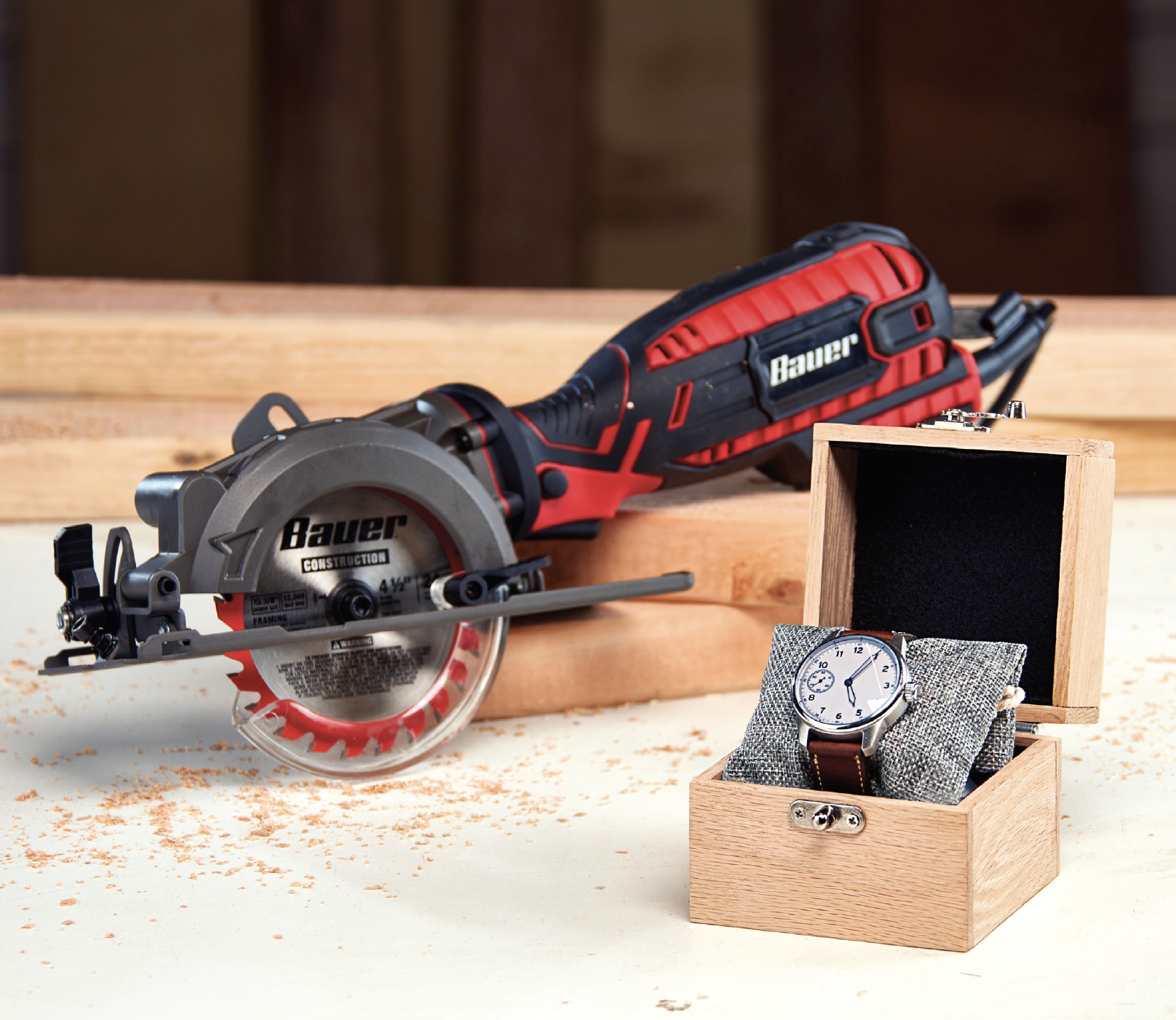In the image, a meticulously crafted wooden box holds a sophisticated brown leather watch, with its silver face prominently displaying regular numerals and a smaller inset dial marking seconds in ten-second increments. The watch is wrapped around a soft, gray cushion, with the inside of the box lined with dark felt. The light, unstained wood of the box has a simple latch, and it sits open on a white surface scattered with wood shavings, indicating recent handiwork, possibly from the planks of wood beside it. Behind this, a striking red and black Bauer table saw, identified by its branding and the '4.5-inch blade' label, rests on the same table. The saw features a silver central blade with an outer jagged edge painted red, suggesting it might be newly purchased or prepared for upcoming carpentry tasks. The overall scene gives the impression of thoughtfully chosen gifts, possibly for someone with a keen interest in craftsmanship and woodworking.